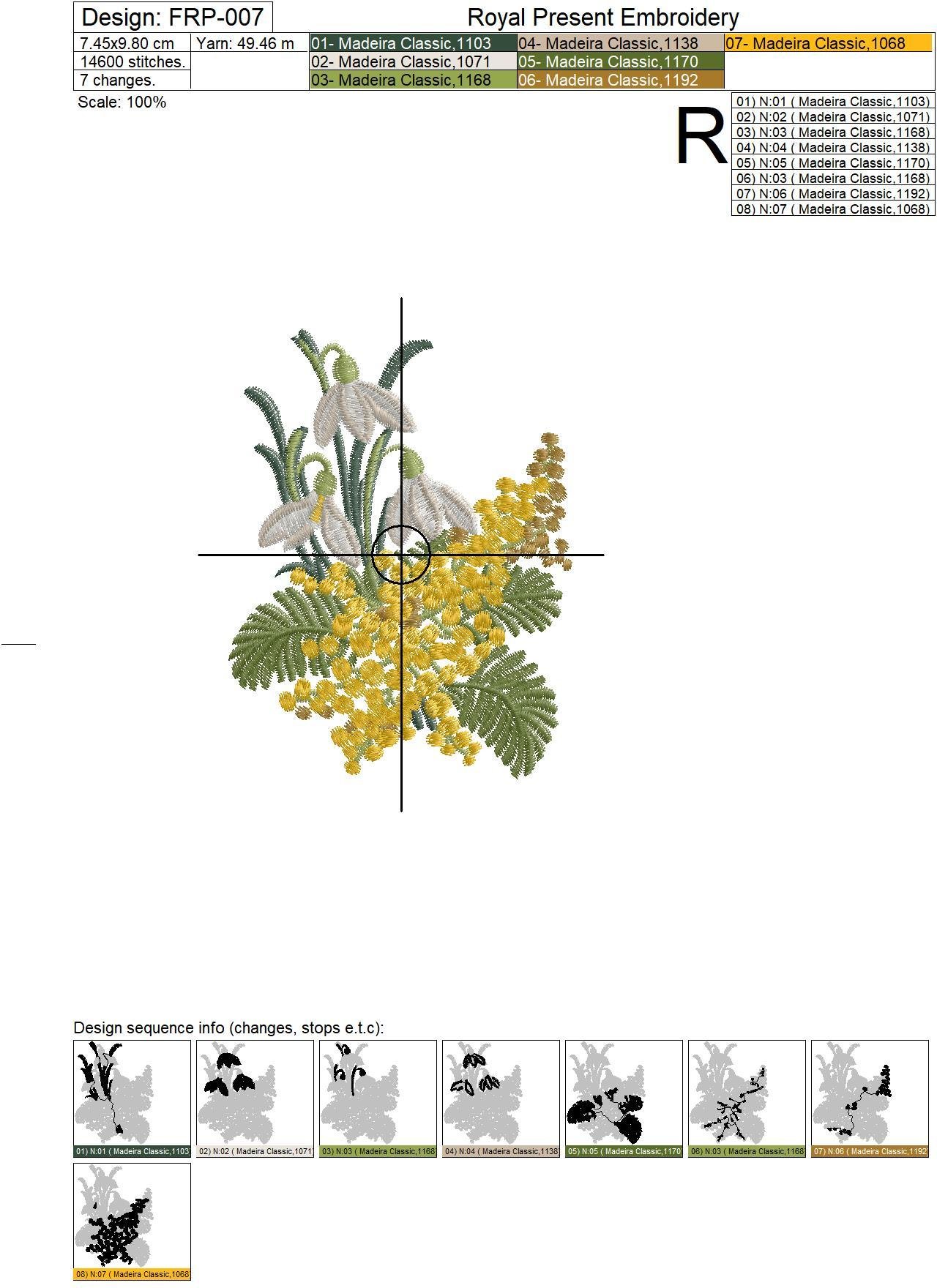The image shows a detailed embroidery pattern generator on a white background, likely captured from a computer screen used for design purposes. At the top, in black text, it reads "Royal Present Embroidery" with the design label "FRP 007" just below. The central illustration is a floral arrangement featuring a green fern-like plant with fan-shaped greenery, adorned with yellow flowers bunched together and white flowers on elongated stems. There's a black crosshair over the plant, likely to indicate the center of the design. The layout includes a three-row by five-column table listing the embroidery specifications: "80 cm," "14,600 stitches," and "seven color changes," along with various thread color codes. At the very bottom, the pattern is outlined with eight segmented squares, showing different stages or sections of the design. This tool appears well-suited for beginners looking to start embroidery, providing all necessary details for creating a 7.45 by 9.8 cm embroidered piece.